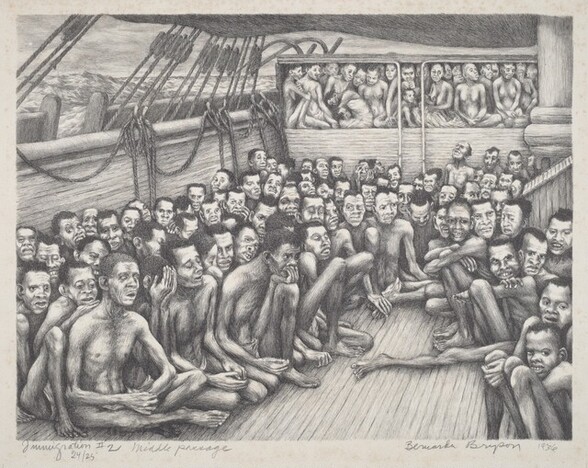The illustration depicts a harrowing scene aboard a slave ship. Rendered in black and white with meticulous shading, the hand-drawn sketch emanates an old-time, historical atmosphere. The ship, constructed of wood with visible rails and ropes, is packed with emaciated African men, women, and children who appear malnourished, their skeletal frames accentuated by the artist's detailed pencil work. These individuals, mostly unclothed, fill every available space, with no room for privacy or comfort. 

The lower deck is crammed with people sitting closely together, their expressions a mix of fear, exhaustion, and despair. You can discern two distinct platforms within the ship: a lower section where the majority of the enslaved individuals are huddled, and an upper deck with additional groups of people, both sections connected by a ladder. The space appears suffocating, a stark representation of the Middle Passage, the horrifying journey where enslaved Africans were transported across the Atlantic Ocean. 

The drawing includes some text at the bottom, partially legible, indicating information about the voyage. Phrases like "Return Number Two, Middle Passage, 24/25," and a name that seems to read "Bermuda Bryson, 1936" can be made out, suggesting it might be a limited print or a documented illustration. This evocative and detailed drawing stands as a powerful testament to the inhumane conditions endured by enslaved Africans during transportation.